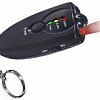The image depicts a small, black device that resembles a car key fob. It's shaped like a long, flat, rectangular piece of black plastic with rounded edges, and features a silver keyring at one end, indicating it's meant to be carried. The fob includes three colored lights—red, yellow, and green—along its top edge, with a red light at the very top. Below these lights, there is a single black button in the middle, appearing to function as a locking mechanism. The top red light is illuminated, and a person's finger is seen poking it, suggesting interaction with another button or switch on the device. The picture, while small and somewhat fuzzy, has a white background and visible white lettering on the device.